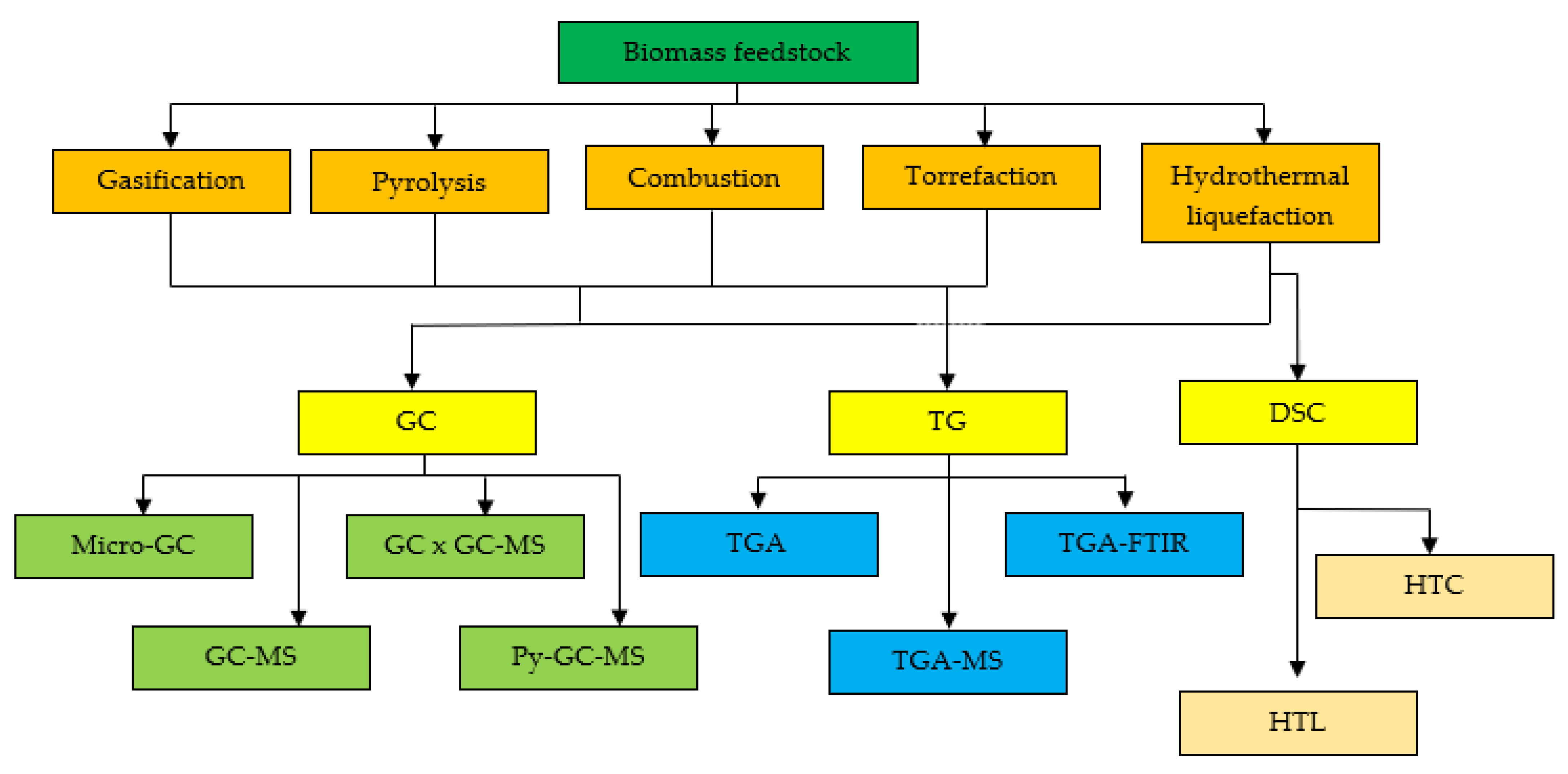The image is a detailed flow chart on a white background, with a green horizontal rectangle at the top titled "Biomass Feedstock." Below this, five orange horizontal rectangles are aligned vertically, labeled from left to right as: Gasification, Pyrolysis, Combustion, Torrefaction, and Hydrothermal Liquefaction. Each of these orange rectangles leads downward via arrows to three distinct yellow horizontal rectangles labeled GC, TG, and DSC. The GC rectangle is further connected downward to four green rectangles on two levels: micro GC, GC-X, GC-MS, and py-GC-MS. The TG rectangle leads down to three blue squares: TGA, TGA-FTIR on the first level, and TGA-MS on a lower level. Lastly, the DSC rectangle flows into two light brown rectangles: HTC and HTL, arranged one above the other. Each label is in black print.